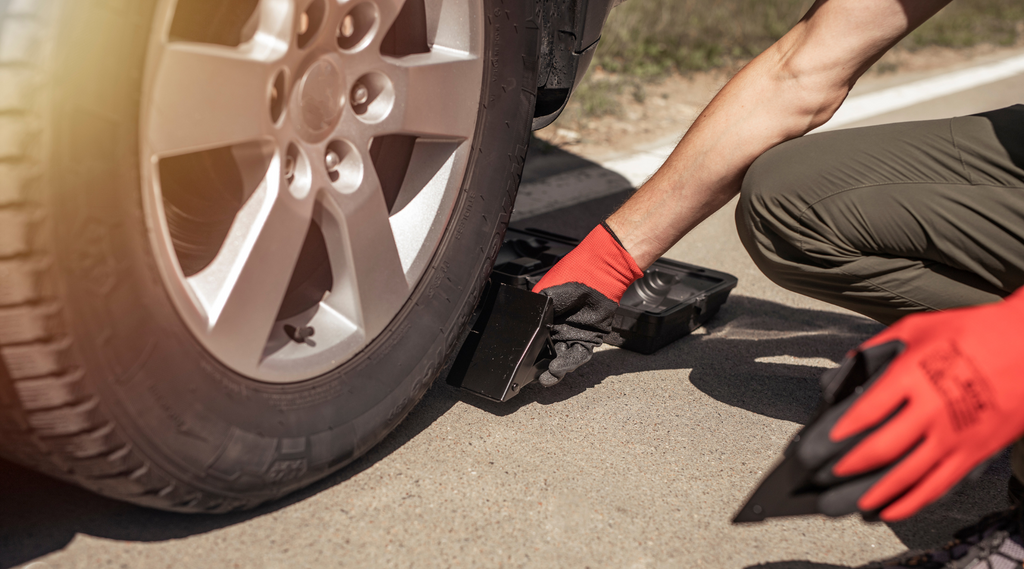In the image, a man is seen bent over, working to secure a black metal wedge beneath a vehicle's tire. The tire has a center silver wheel hub with six nuts and a visible valve positioned at the bottom. The man, dressed in olive-colored pants and grayish tennis shoes, is wearing black and red neoprene gloves on both hands. His exposed, lean arm is not very hairy. Additionally, his left hand is holding a blurred triangular object, possibly to aid his efforts. The setting is a sunny roadside, marked by a white reflective stripe and bordered by scrub brush and grass. Behind the tire, an open toolbox or tray is visible, suggesting that the man is either fixing the tire or preparing for a potential tire change.